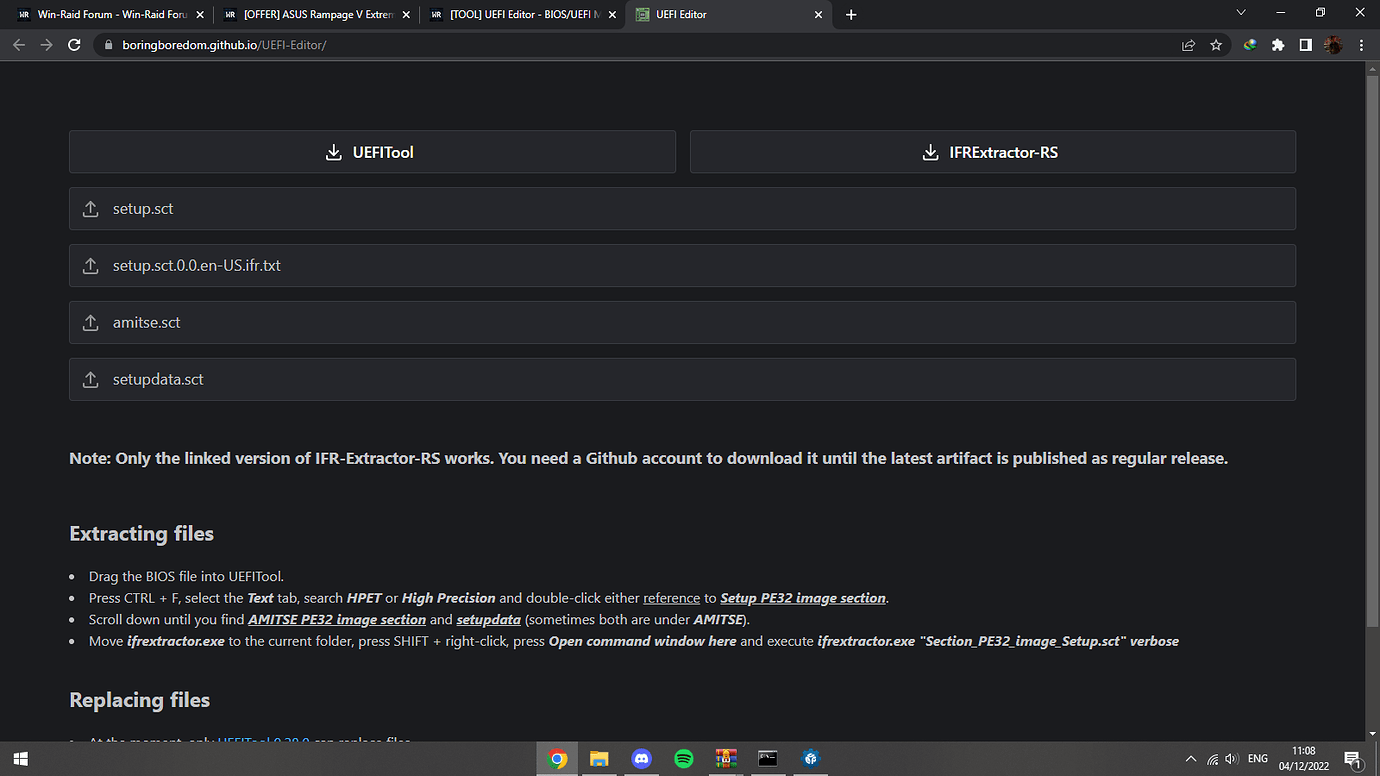The image captures a computer screen displaying a GitHub webpage dominated by a dark black color scheme with white text. At the top of the page, the title reads "Boring Boredom - GitHub.in". The navigation area beneath the title includes clickable sections for easy access. In the bottom-right corner, additional icons are available for further interactions.

The central portion of the screen features two prominent download links labeled "UEFITool" and "IFRExtractor-RS." Adjacent to these downloads are a series of four upload buttons positioned along the left side of the page. Below this, a notable line of white text reads: "Note: Only the linked versions of IFR-Extractor-RS work. You need a GitHub account to download it until the latest artifacts are published as a regular release."

At the bottom, the page provides detailed instructions on extracting and replacing files, ensuring users have the information they need to proceed with their tasks on the site.